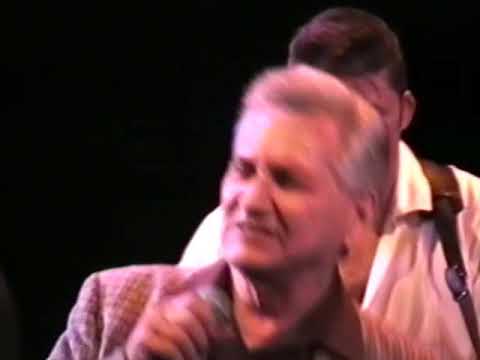The image depicts a somewhat grainy and blurry photograph of two men standing against a pure black background, with an orange tinge affecting the coloration. In the foreground, there is a white-skinned older gentleman, likely in his early 40s, with silver-gray hair swept back on the sides and slightly fuzzy on top. He is dressed in a tweed sports jacket and a brown collared shirt. This man appears to be leaning slightly to the left, facing the camera with a microphone in his right hand, which is positioned to the left in the image.

His face is slightly pink, with recessed lines along the sides of his nose and lips that are partially open. Standing directly behind him is a younger man with dark brown hair, wearing an open-collar white button-down shirt. A brown strap, likely for a guitar, runs over his left shoulder. Both figures are captured indoors, and the photograph measures approximately three inches wide by two inches tall.